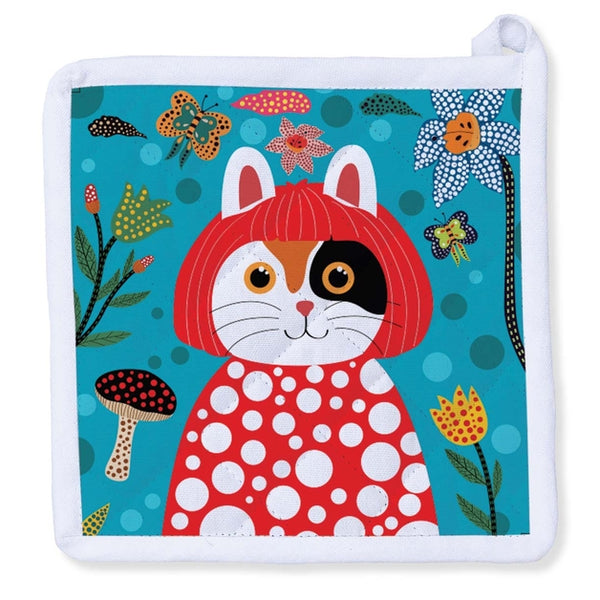The image depicts a colorful, animated square rendering of a cat with human-like attributes. The cat, predominantly white with a black patch around its left eye and an orange forehead, has a red nose and a small smile. It wears a short red wig, giving it a unique and vibrant appearance. The cat dons a red and white polka-dotted shirt that obscures its arms and paws. Surrounding the cat, the aqua blue background is embellished with an assortment of polka dotted flowers, including blue and yellow blooms, a green tulip on the top left, and variously colored butterflies flitting about the scene. Mushrooms also stem from the green tulip, adding to the whimsical nature of the artwork. The entire piece is framed by a white border, with the top right corner slightly rolled up, contributing to the charm of the illustration.